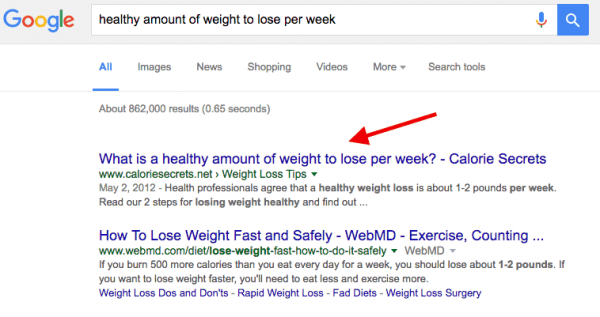**Detailed Caption:**

The image displays a Google search results page. In the upper-left corner, the iconic multi-colored "Google" logo is prominently visible. The search bar contains the query, "healthy amount of weight to lose per week." To the right of the search bar, there's a small microphone icon for Google voice search, and a blue search button next to it.

Below the search bar, several navigation options are displayed, with "All" highlighted in blue. Other options like "Images," "News," "Shopping," "Videos," "More," along with a dropdown menu for "Tools," appear in gray. Additionally, the phrase "About 862,000 results (0.65 seconds)" is shown, also in gray.

A red arrow points downward to the first search result, which is titled, "What is a healthy amount of weight to lose per week - Calorie Secrets," in blue text. Below the title, the URL "caloriesecrets.net" is displayed in green, followed by a snippet of the article summary. The summary reads, "May 2nd, 2012 - Health professionals agree that a healthy way to lose weight is about 1-2 pounds per week. Here are two steps to losing weight healthily and find out more.”

The next search result begins with the query "how to lose weight fast and safely - WebMD," followed by a truncated URL "WebMD.com/diet/lose-weight-fast-how-to-do-safely." The snippet within this search result states, "If you burn 500 more calories than you eat every day for a week, you should lose about 1-2 pounds. If you want to lose weight, eat less and exercise more." Additionally, there are blue hyperlinks including "Weight loss do's and don'ts," "rapid weight loss fad diets," and "weight loss surgery."